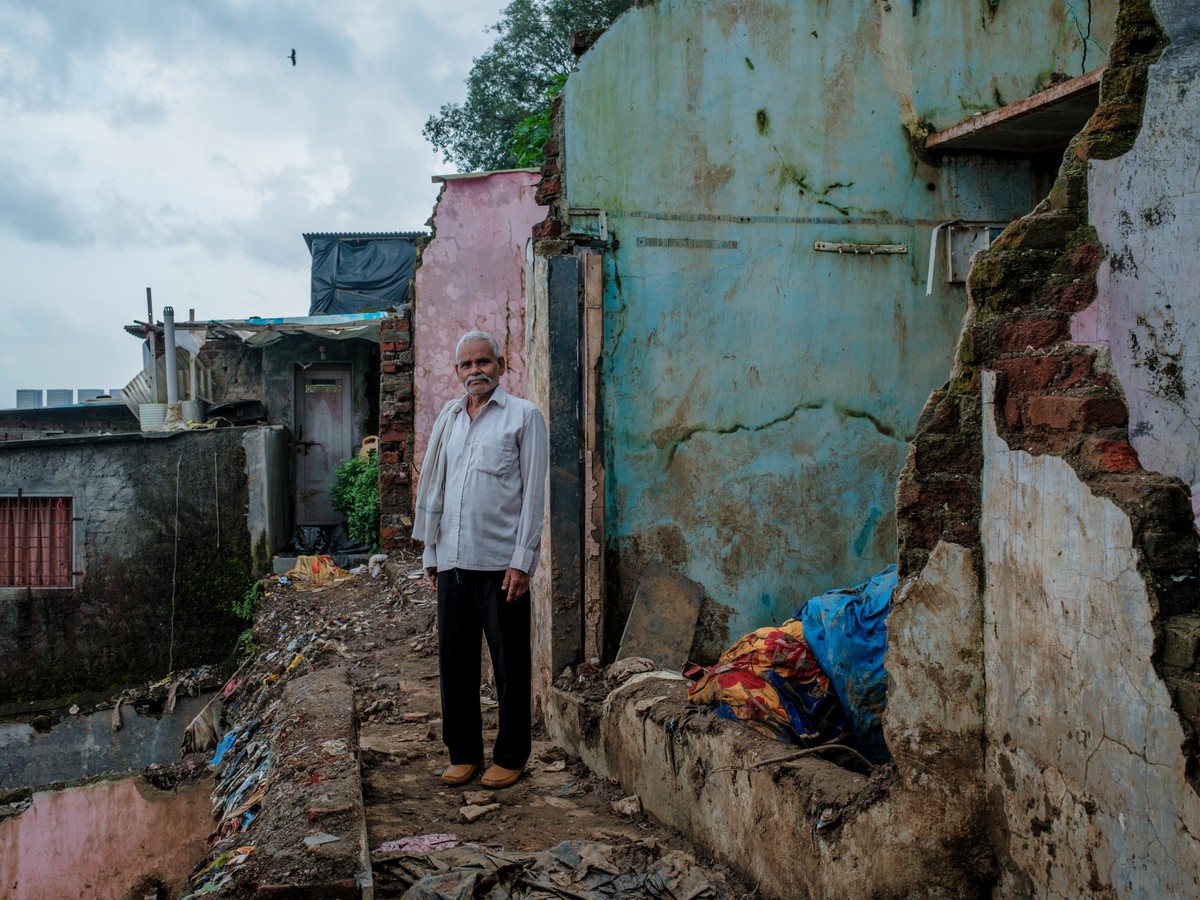This photograph vividly captures an elderly man, likely in his late 60s or early 70s, with a medium to medium dark complexion, short gray hair, a gray mustache, and dark eyes. He is wearing a white long-sleeve shirt that is slightly unbuttoned at the top, black pants, and brown shoes. Draped over his right shoulder is a towel or cloth. He stands amidst the ruins of what appears to be a slum or an area that has faced severe destruction. The background showcases buildings that are heavily damaged, with crumbling and exposed brick foundations, some parts with vegetation growing over them, indicating long-term neglect. The sky is cloudy, and above his left shoulder, a bird is seen flying. A prominent feature in the backdrop is a cracked blue wall, with dirt and debris scattered around. The lower part of the building shows multiple colors, including signs of a yellow and red image and areas painted in blue and pink. The overall scene conveys a sense of desolation and enduring hardship.